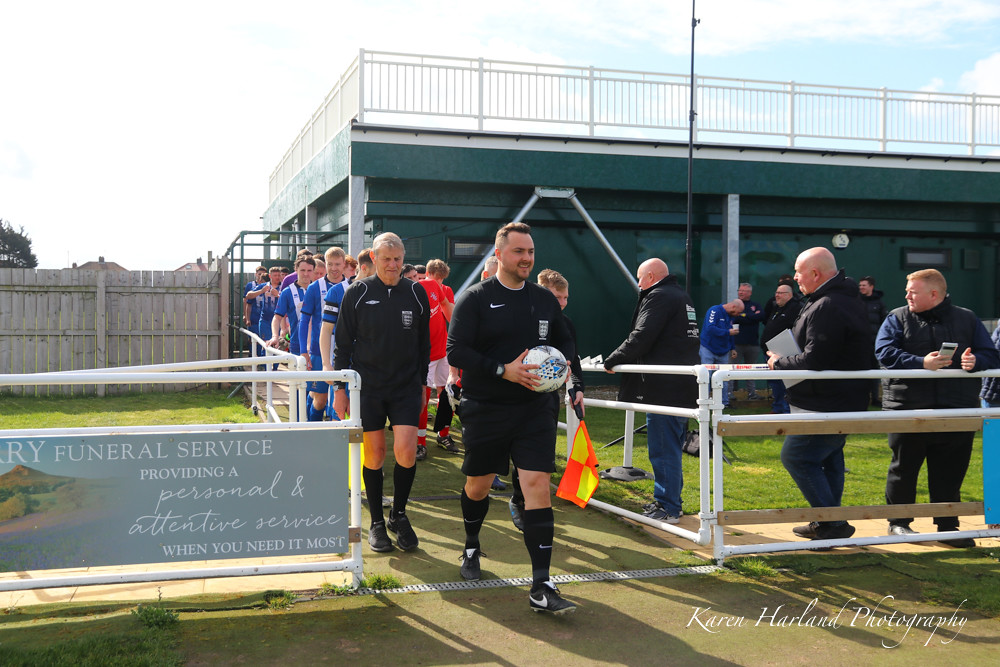This detailed image captures a moment outside a soccer stadium where multiple soccer players are preparing to play. They are seen walking through a white PVC pipe gate onto a grassy path, with a backdrop of a green building topped with a fence. Leading the group is a man in an all-black Nike uniform, short brown hair, and holding a white soccer ball with blue accents. Another player in identical attire follows him closely. Behind them, several players wear a mix of blue and black jerseys, some in long-sleeved blue shirts, and there’s a distinct player in a red and white jersey, matching white shorts, and red knee pads. All players are equipped with mostly black cleats. 

Spectators, including two bald men in black jackets, stand outside the fence, observing the procession. One is engaged in conversation, holding a notebook or some papers, and another with a phone in hand, appears to be watching the players. The sky above is mostly blue, and the sun lights up the scene, indicating it's daytime. A sign near the gate reads, "Funeral Service: Providing a personal and attentive service when you need it most." Additionally, "Karen Harland Photography" is noted in white letters at the bottom right of the image.